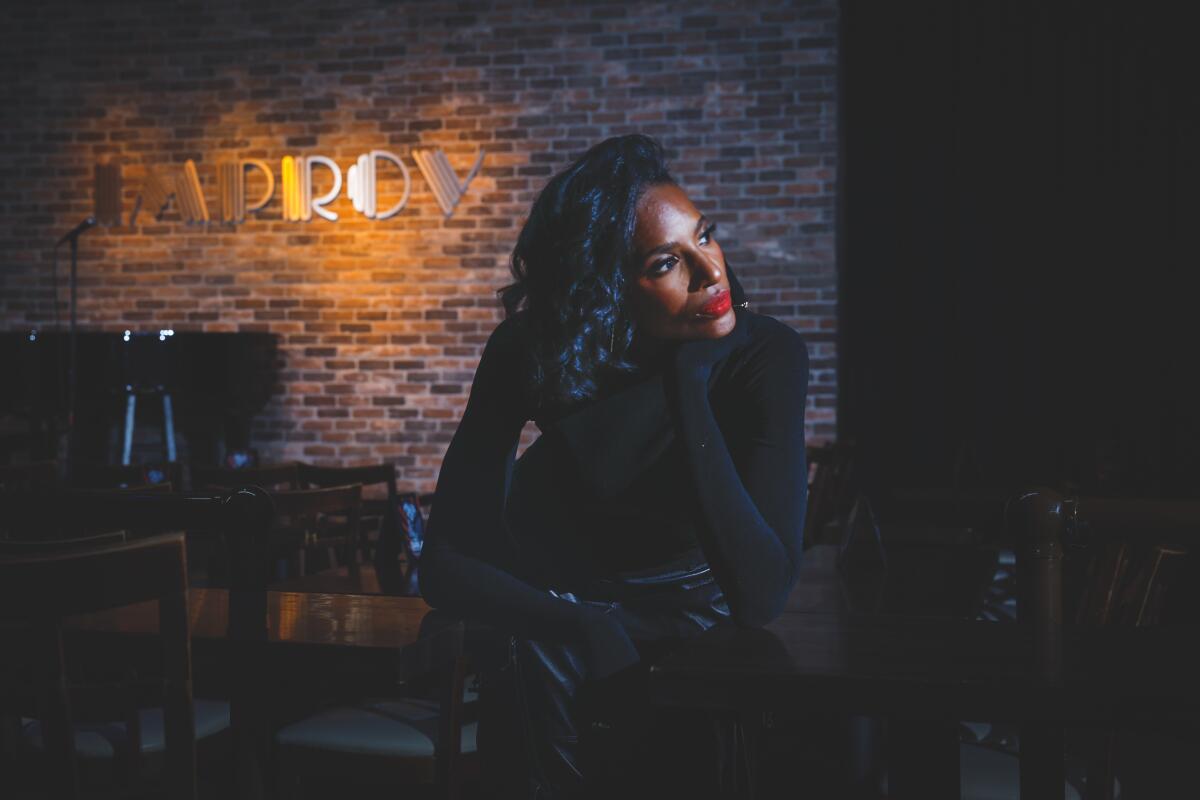The photograph is a dimly lit image taken indoors, capturing a moment with a distinct ambiance reminiscent of a dive bar. Central to the scene is an African descent jazz artist seated at a table. She occupies the middle of the frame, her body angled towards the camera while her head turns to the right. Her left hand supports her chin, with her elbow resting on the black shadowed table. Her right arm is relaxed on her knee. She wears a seamless long black shirt with matching gloves, paired with black leather pants, and accentuates her look with bright red lipstick.

The background features a brick wall on the left adorned with a spotlight illuminating the word "improv." Positioned in the backdrop, there’s a piano and stage, typically left of center. Surrounding this area are numerous seats, indicative of an intimate performance space. The color palette comprises various dark tones including brown, black, brick red, and shades of dark brown, enhancing the intimate, moody atmosphere of the bar. To her left, another table is visible in a dark brown hue, further deepening the cozy, shadowy environment. The photograph's dimensions are roughly six inches wide by three inches high, emphasizing the elongated rectangular shape.